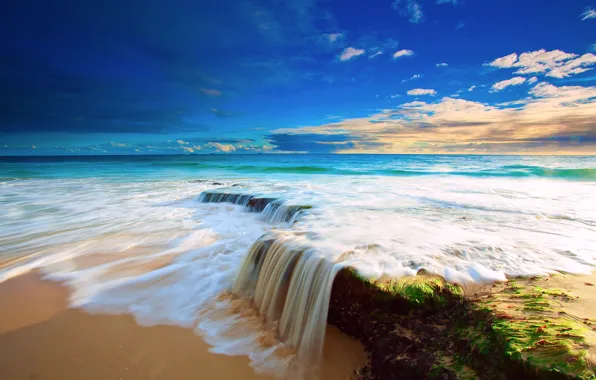This image is a highly detailed and vibrantly colored 3D rendering in landscape orientation, capturing a beautifully surreal beach scene during the daytime. The shoreline extends horizontally across the center, featuring gentle waves that come ashore with white foam, which contrasts strikingly against the pinkish-beige, almost orange-colored sand in the foreground.

To the right, a rocky outcropping adorned with green moss adds texture and depth. This outcropping angles towards the center of the image and features a small, yet picturesque waterfall created by the waves crashing over it. The waterfall appears straight and somewhat blurred, suggesting a motion captured in a long-exposure shot, blending seamlessly with the white foam below.

The ocean water transitions from a near-shore aqua blue to richer turquoise and finally to a deep, rich blue in the distance. Above, the sky is a dark, intense blue interspersed with large, rolling white clouds, through which the sun beams, illuminating the entire scene with a dreamy quality. Together, these elements create an exquisitely detailed and captivating depiction of a beachscape.